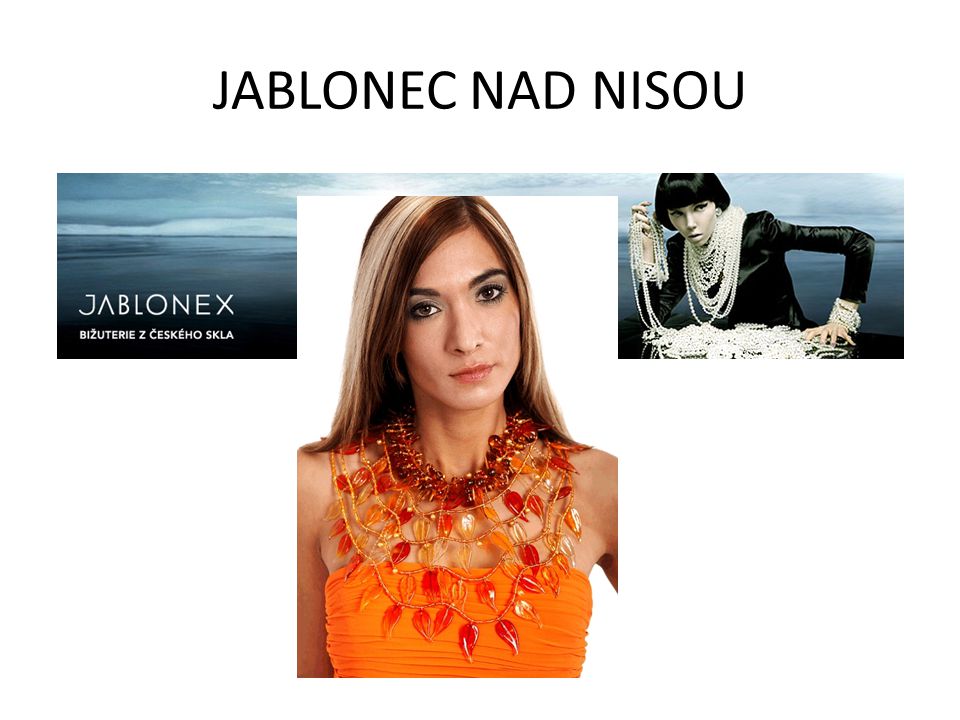This image appears to be an advertisement from the Czech Republic or an Eastern European country, prominently featuring the text "Jablonec nad Nisou" at the top. The advertisement is divided into three sections with different photographs and details.

On the left, an image portrays a serene ocean scene with a dark cloud stretching across a light sky. Overlaid on this backdrop is white, stylized text spelling "Jablonex," followed by additional foreign text.

The center of the advertisement highlights a light-skinned model with shoulder-length brown hair streaked with white. She has a calm expression with her mouth closed, wearing an elaborate multi-strand necklace adorned with red, teardrop-shaped pendants. Her outfit consists of a yellow-gold, shoulderless top or dress that complements the necklace.

On the right, a second woman is prominently featured, dressed in a black long-sleeved outfit and adorned with numerous strings of pearls. She poses with pearls wrapped around her arm and scattered on the table in front of her. Her dark, pixie-cut hair frames her face as she gazes directly at the camera.

Collectively, the advertisement showcases a blend of elegant and artistic imagery, focusing on the sophisticated display of jewelry, particularly necklaces and pearls.